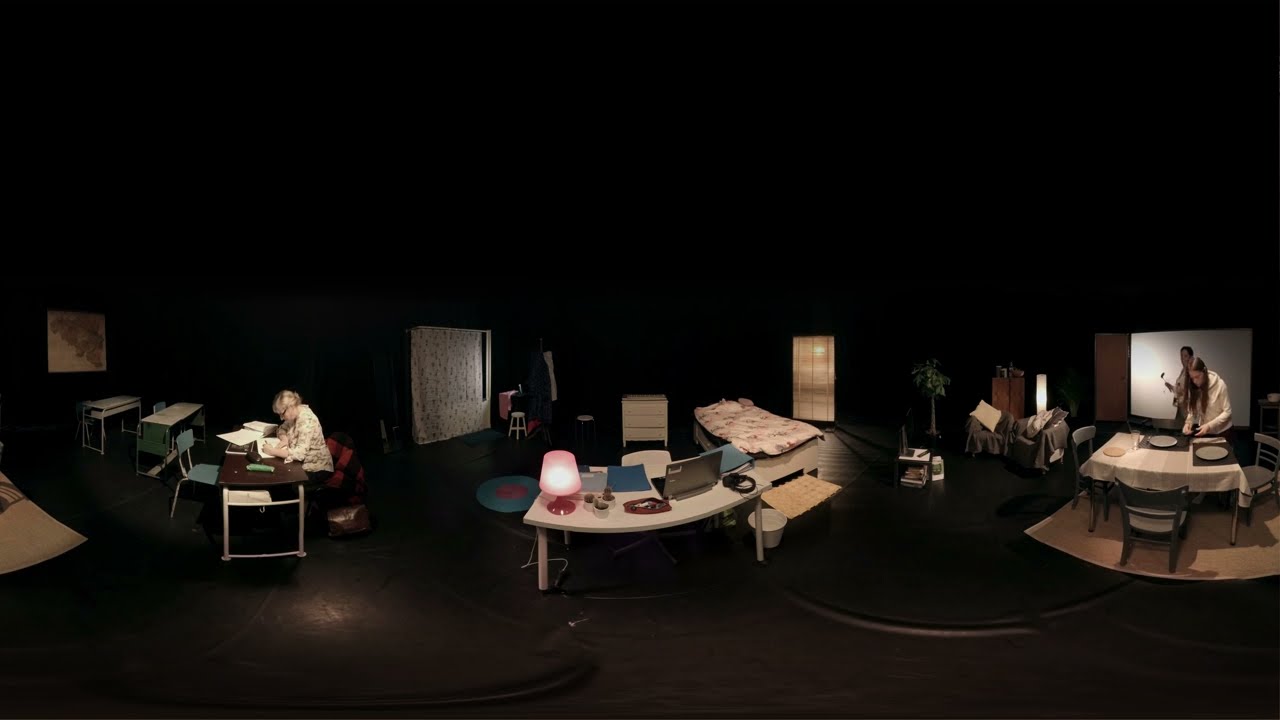The image portrays the interior of a dimly-lit room, potentially a conference or convention setup. The room features several tables arranged in a curved layout, each adorned with laptops, notebooks, various paperwork, and lamps. The tables are light tan in color, and the floor is a dark brown shade that contrasts with the pitch-black background. Behind each table, large white screens prominently display emblems resembling blue diamonds with sunset hues of blue and orange, possibly serving as logos or informational displays. The front of these signs is white, with a blue top section, enhancing their visibility. Two women are present on the right-hand side, one standing in front of a table and the other behind it, both seemingly focused on their tasks, with one looking at a phone. The overall ambiance suggests a professional yet mysterious environment, possibly an office area, a banquet setup, or a conference space.